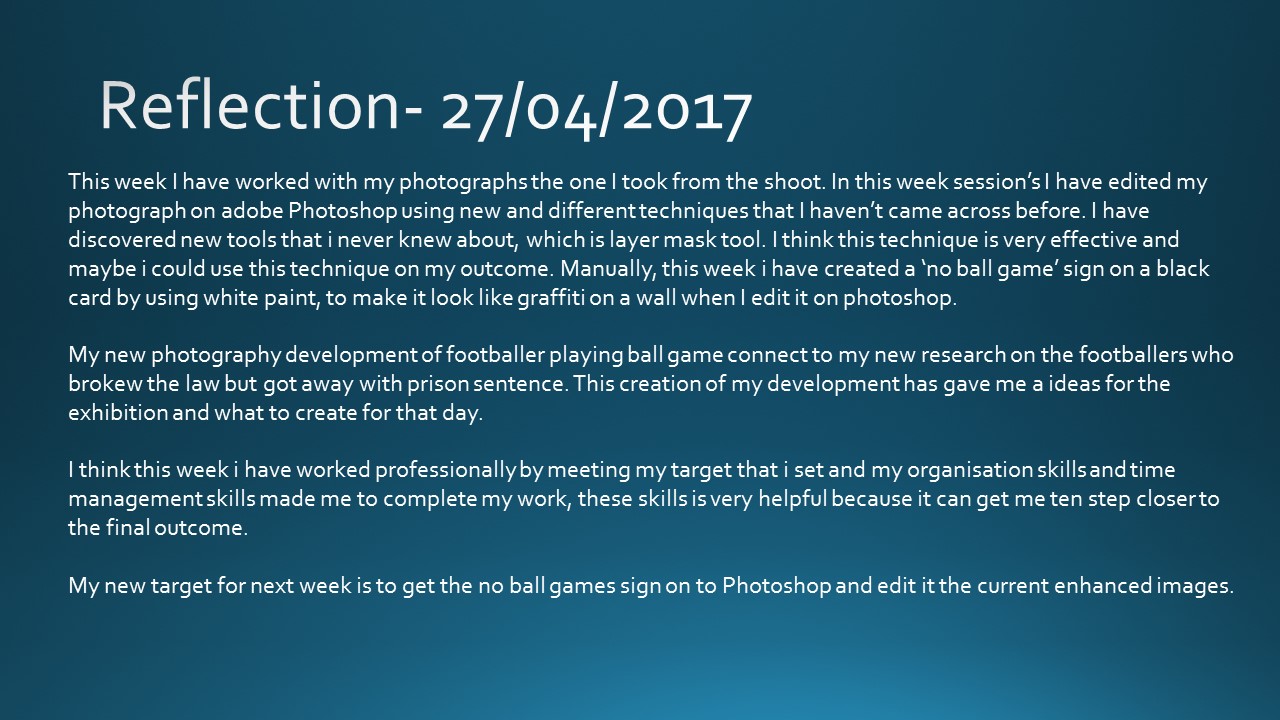The image appears to be a screen capture resembling a diary entry, set against a dark blue background that fades to a lighter shade towards the bottom. The title "Reflection-27-04-2017" is displayed at the top in white text, indicating a date of April 27, 2017, using the European date format. The content is organized into four paragraphs.

In the first paragraph, the author, a photographic artist, reflects on their week's work, mentioning that they have edited photographs from a recent shoot using Adobe Photoshop. They highlight the use of new techniques and tools, specifically the Layer Mask tool, which they found to be very effective and consider applying to future projects.

The second paragraph discusses a manual creation process where the artist made a "no ball games" sign using white paint on black card to resemble graffiti. They plan to incorporate this into their edited photographs in Photoshop. 

The third paragraph connects the new photography developments to the artist's research on footballers who have had legal issues but avoided prison sentences. This research has inspired ideas for an upcoming exhibition.

In the final paragraph, the artist reflects on their professionalism, citing successful achievement of targets due to good organization and time management skills. These skills are deemed crucial for getting closer to their final outcome. Their new target for the following week is to integrate the "no ball games" sign into their enhanced images in Photoshop.

Overall, the entry showcases the artist's workflow, creative processes, and aspirations, albeit with grammatical imperfections indicative of a non-native English speaker.